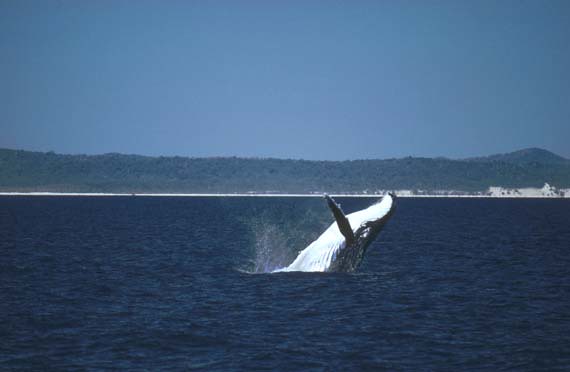In the image, a magnificent blue whale is captured breaching in the middle of a calm, deep navy blue ocean. The whale's underbelly, painted a stark white, contrasts sharply with its dark blue back. One of its fins is visible, dark in color, gracefully arcing upward as it makes a gentle splash. The whale appears to be leaning its head back out of the water, creating a dramatic yet serene moment.

The ocean itself is a rich, highly pigmented dark blue, extending to a distant white horizon that blends into a flawless deep blue sky. There are no clouds or sun visible, emphasizing the clarity and tranquility of the scene. Beneath the horizon, a steady plateau of land spans from left to right, covered with bushy trees and punctuated by a small hill or mountain on the right-hand side. A sliver of a beach is also perceptible, adding to the lush and textured backdrop of this captivating marine vista.